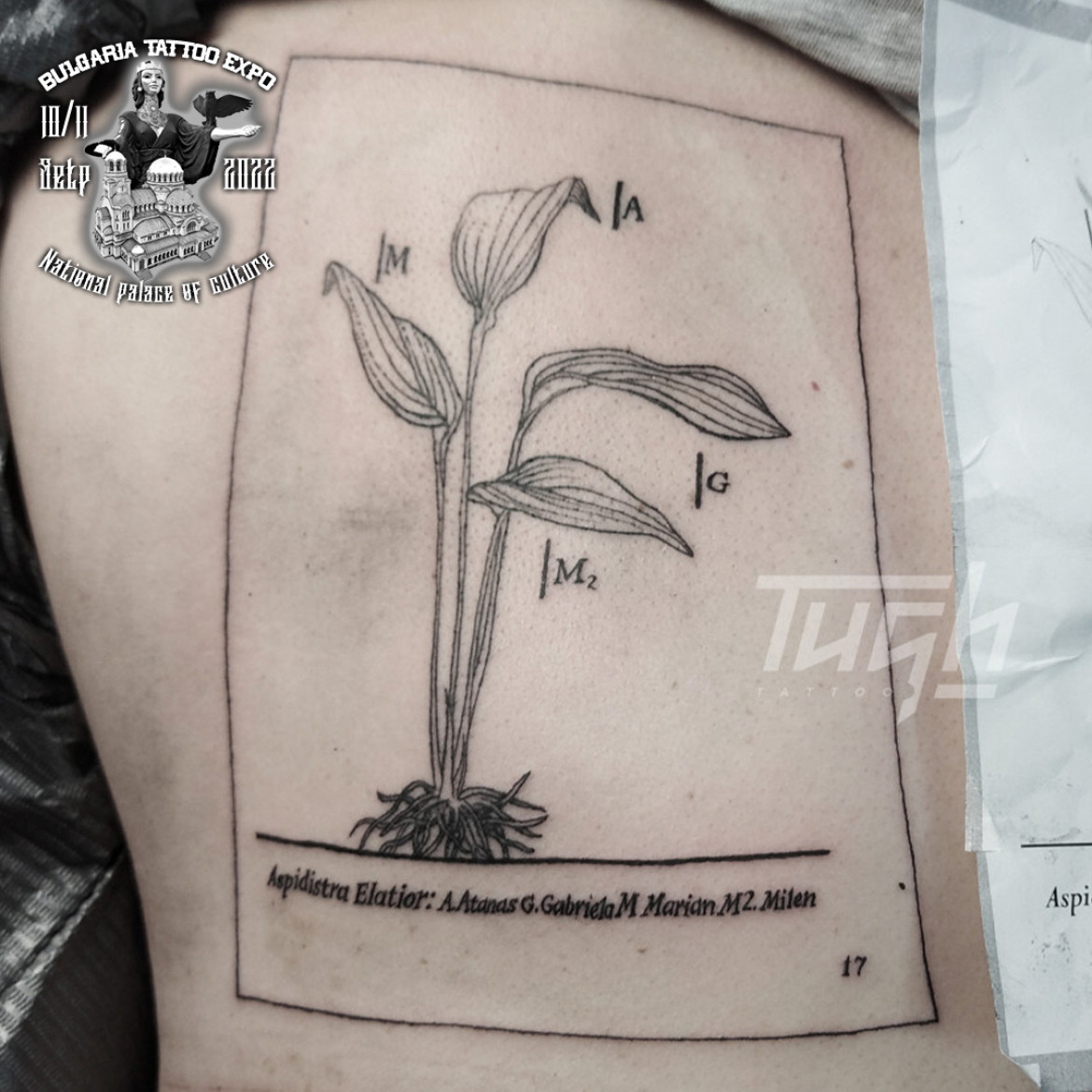The image depicts an advertisement for the Bulgaria Tattoo Expo held at the National Palace of Culture on October 10-11, 2022. In the top left corner, there's a logo featuring a woman, possibly adorned with a crown and a black dress, holding out her arm with a crow or similar bird perched near her elbow. The central element of the tattoo itself is a detailed illustration resembling a science textbook page. It features four leaves labeled 'M,' 'A,' 'G,' and 'M2,' with roots extending beneath a line that likely represents the ground. Below the botanical illustration, the text reads "Aspidistra Elatior," followed by a series of names and the number 17, indicating it might be from page 17 of the referenced book. The tattoo is framed by a thin black line and is depicted on an indistinguishable part of the skin, making it difficult to determine its exact location on the body.